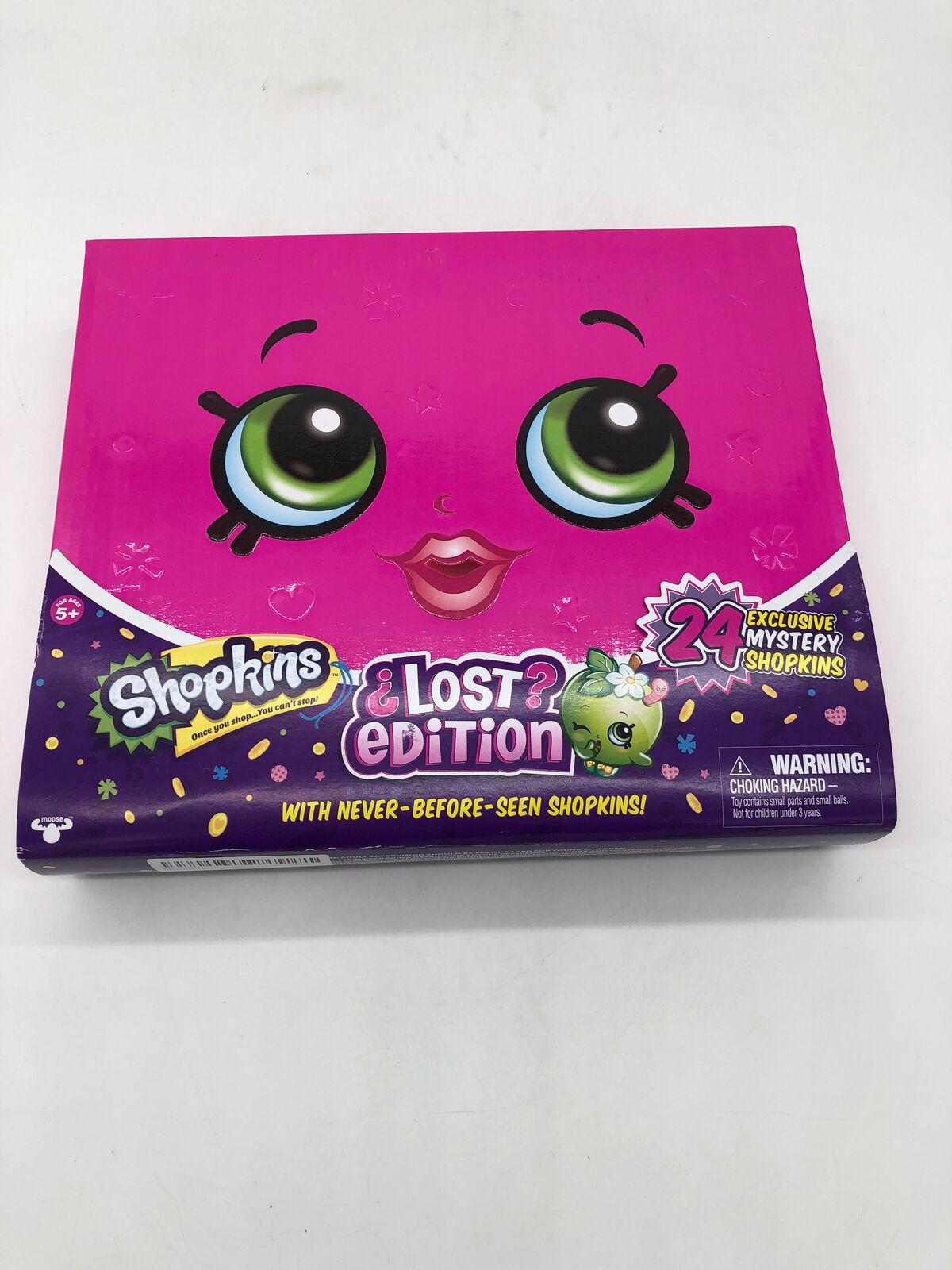This is a detailed photograph of a children's toy package set against a white background. The package features a predominantly bright pink area that covers the top two-thirds, transitioning into a white banded curve near the bottom, and finally into a deep purple color for the remaining lower portion. The top pink section displays a cartoon-style face with distinctive green irises outlined in black, looking up and to the right. The face also includes arched black eyebrows above the eyes and stylized pink lips positioned in the center.

On the purple lower section, various logos and text are prominently featured. To the left, the logo "Shopkins" appears in playful white cartoony text against a green and yellow backdrop. Adjacent to this logo, in blocky white text with a pink gradient, it reads "Lost Edition," flanked by an upside-down question mark preceding "Lost" and a right-side-up question mark following it. To the right of this text, a green cartoon apple character with a pink worm emerging from its head is visible. Slightly above and further to the right, bold text announces "24 Exclusive Mystery Shopkins," with "24" in vibrant pink, set against a purple burst, while "Exclusive" and "Shopkins" are in yellow, and "Mystery" is in white. Toward the very bottom of the package, additional yellow text declares, "With Never Before Seen Shopkins."

In the bottom right corner, there is a pale white-outlined box that carries a safety warning: "Warning Choking Hazard. Toy contains small parts and small balls. Not for children under 3 years." On the bottom left, a stylized white moose symbol is present, accompanied by the word "Moose" in white text above it.